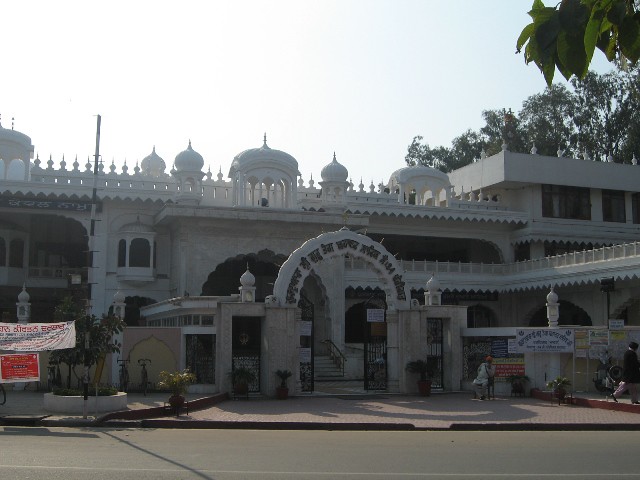The photograph captures the front of a large, older-style rectangular white building, located outdoors on a bright day with a clear light blue sky above. In the top left corner, the sun is visible, casting a significant glare on the camera lens. The top right corner of the image is adorned with branches of leafy green trees that frame part of the building. At the forefront, a smooth, black asphalt road with a white line runs horizontally, indicating either a lane or edge. Just beyond the road, there's a sidewalk where people can be seen walking around, and bicycles are parked, enhancing the scene’s activity and urban feel.

Dominating the center of the image is the building, which features various stone spikes along its edges and railings. The large arched entrance gate, made of open wrought iron fences, leads into the building. Above this gate, there are steeples, with Asian symbols and writing adorning the archway and entrance. Additional signs with Asian or Chinese characters can be seen on the far left and right sides of the entrance, possibly indicating advertisements or promotional material. The entire scene is a harmonious blend of architectural elements and natural surroundings, painted in hues of white, off-white, green, red, orange, tan, and black.